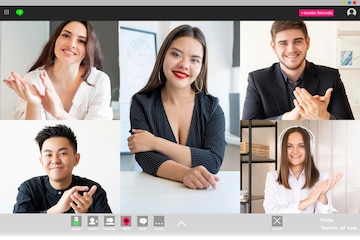This is an image of a video conference call featuring five participants displayed on what appears to be a computer screen, evidenced by the visible screen controls and app icons at the top and bottom edges. The display is divided into five sections. 

In the top left corner is a young Caucasian woman with long black hair, wearing a white V-neck shirt. She appears to be between 18 and 25 years old. Directly below her, in the bottom left corner, is an Oriental man, also smiling, with short black hair and wearing a black shirt.

Occupying the center column of the screen is another Caucasian woman who seems to be the host. She is seated at a white desk, wearing a three-quarter sleeve black V-neck top. She has long brown hair, hoop earrings, and is visible with red lipstick. A large white bulletin board is seen in the background. Her left arm is cupped around her right arm in a relaxed posture.

In the top right corner, a Caucasian man is seen wearing a black sport coat over a dark gray shirt. He has short dark brown hair and a bit of a beard, and something can be seen hanging on the wall behind him. Finally, the bottom right corner shows a woman in a white long-sleeve blouse with white headphones on. Behind her, a black shelf with folders is visible. Both the man on the top right and the woman on the bottom right have their hands in front of them.

All the participants are smiling, with notable details such as the black clothing theme, the varied backgrounds, and the apparent engagement in a conference call setting.